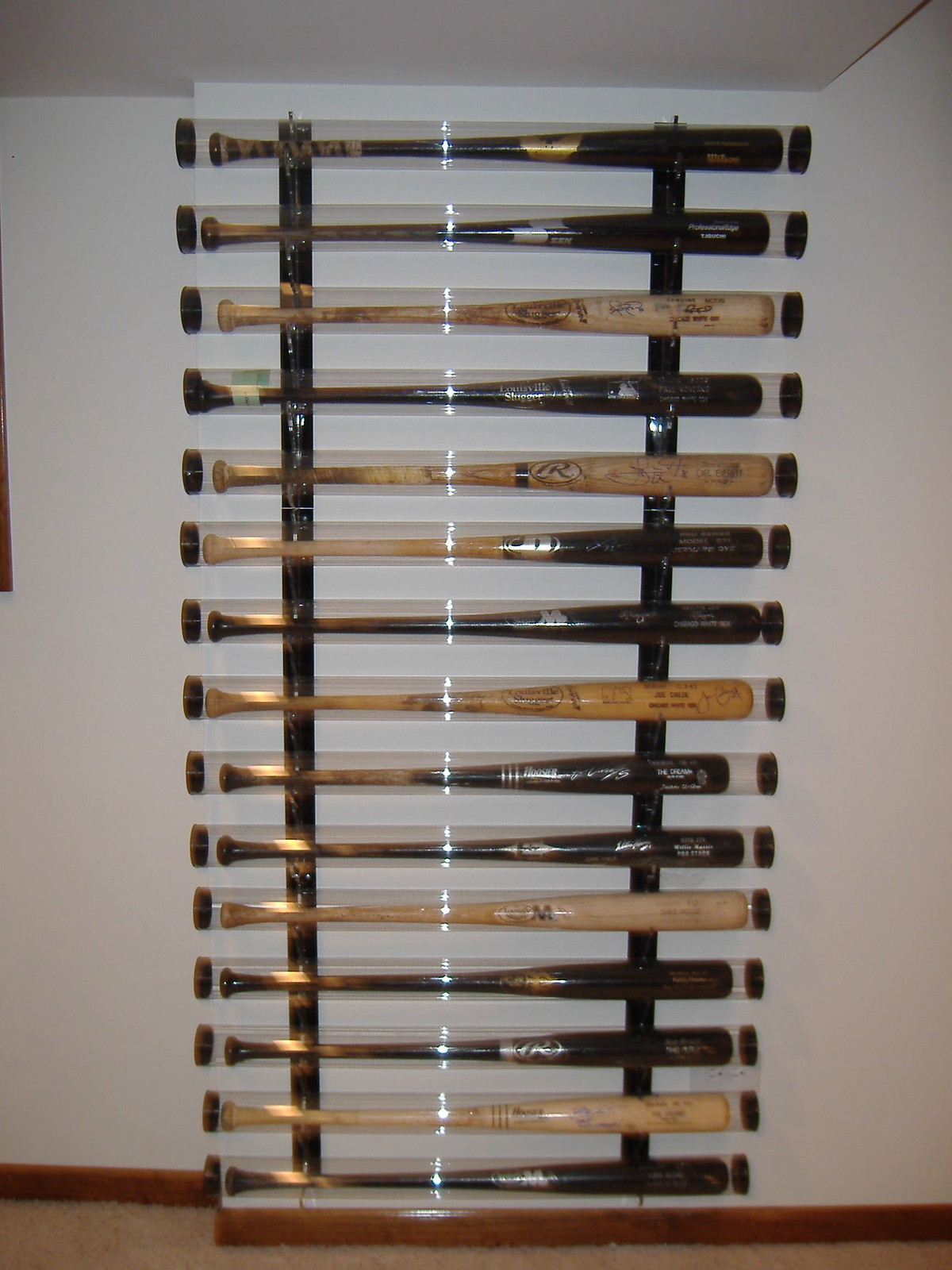This photograph showcases a meticulously arranged collection of 15 baseball bats displayed in individual clear plexiglass or plastic tubes, each sealed with black caps on either end. These tubes extend vertically from the floor to the ceiling, supported by vertical black lacquered wooden braces. The arrangement ensures that while the bats are neatly organized, they remain untouchable and well-preserved, highlighting their likely high value. Many of the bats feature signatures, suggesting they are collectible memorabilia from various Major League Baseball players or teams. The bats come in different styles and brands, including Rollins and Wilson, with color variations ranging from black with silver accents to light beige wood. The display is set against a white wall, complemented by a white ceiling, brown wood baseboards, and tan carpet flooring. The reflective quality of the plexiglass under the overhead light adds a polished and professional touch to the presentation.